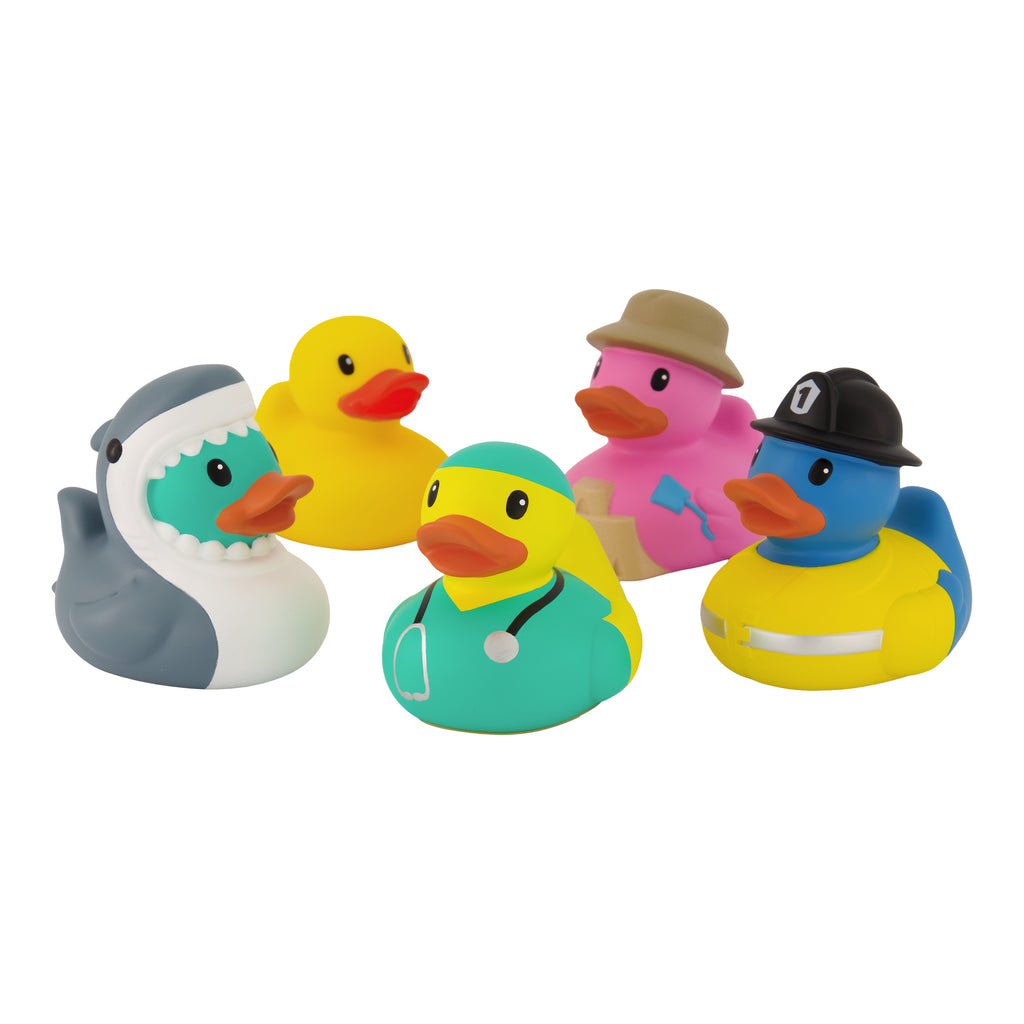The image is a color photograph in landscape orientation featuring five distinct rubber duckies arranged in a circular layout against a white background. In the front row of three, on the left, there's a green rubber duck dressed in a gray and white shark suit with its mouth open. At the center is a yellow rubber duck adorned in teal medical scrubs, a matching cap, and a stethoscope around its neck, looking slightly upward and to the left. To the right in the front row is a blue rubber duck wearing a yellow firefighter suit and a black hard hat, marked with a number one, facing the center. On the back row, to the left, sits a standard yellow rubber duck with an orange beak. Next to it, on the right, is a pink rubber duck in front of a sandcastle, wearing a beige hat and holding a blue sand shovel. The ducks are represented in a photo-realistic style, appearing to float against the pristine white backdrop.